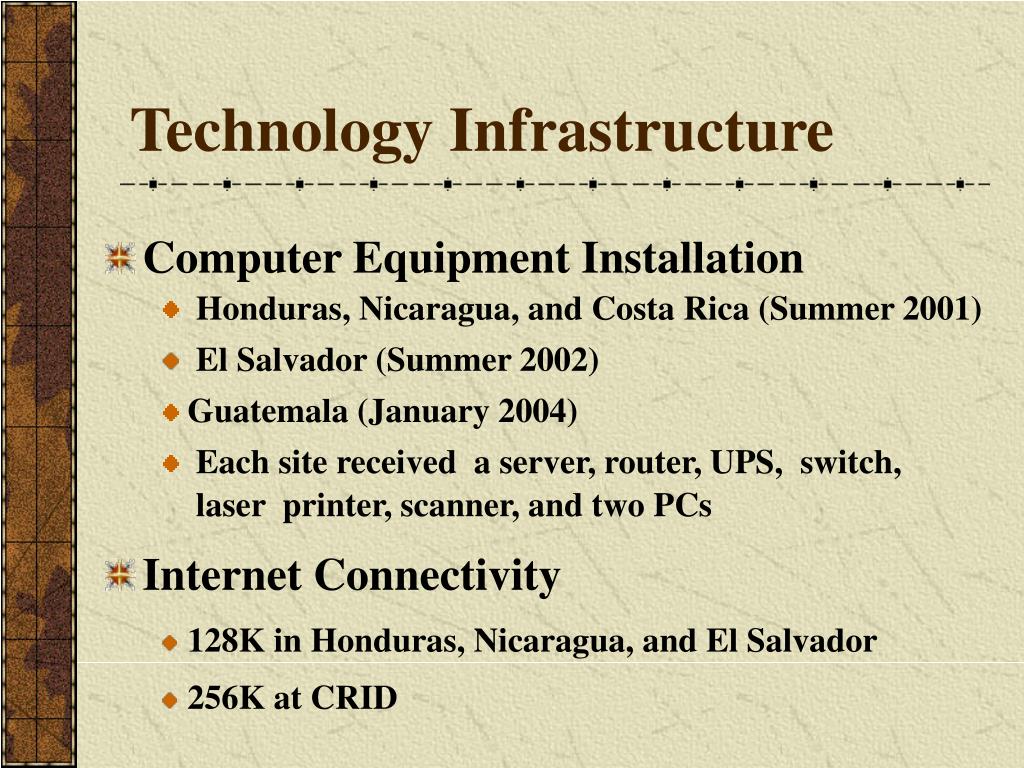The image resembles a page from a pamphlet with a beige background featuring subtle gray lines and speckles. Along the left side runs a brown column adorned with a cream-colored dashed pattern. At the top center, the title "Technology and Infrastructure" is prominently displayed in brown text, followed by a dividing line. Below, there are two main sections of text in black. The first section, titled "Computer Equipment Installation," details several locations and corresponding dates: Honduras, Nicaragua, and Costa Rica in summer 2001; El Salvador in summer 2002; and Guatemala in January 2004. Each site reportedly received a server, router, UPS, switch, laser printer, scanner, and two PCs. The second section is titled "Internet Connectivity" and notes 128K connectivity in Honduras, Nicaragua, and El Salvador, with 256K in Costa Rica. The text uses distinct brown and black colors to highlight the titles and information.